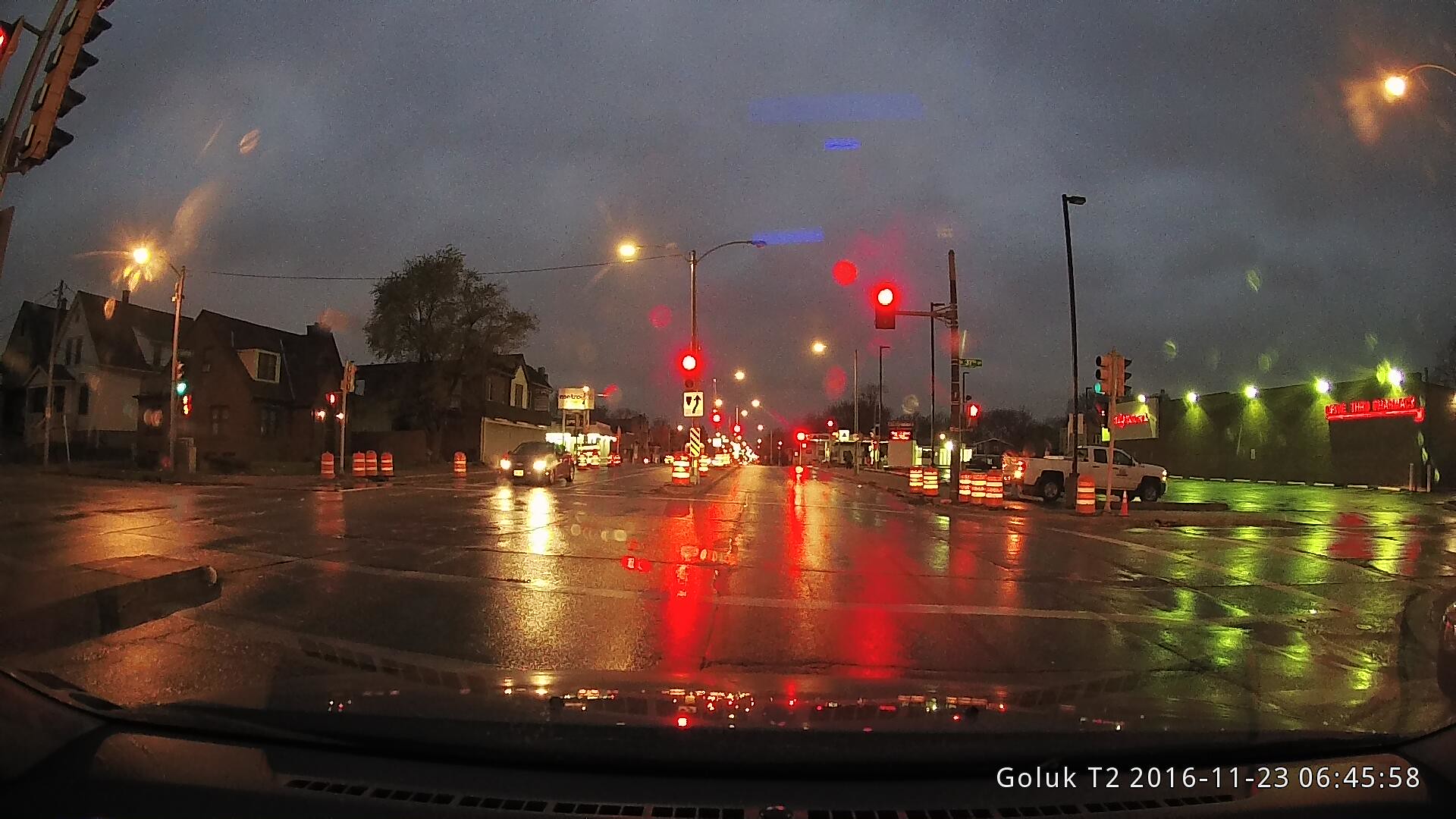The photograph, taken through the windshield of a car, likely using a dashcam, captures a rainy night scene with a dark blue-gray sky. The wet, glistening road reflects the red lights from two traffic signals—one positioned in the upper right and the other in the center of the road. The right-hand side features orange and white striped construction barrels. A building with a bright red illuminated sign and white lights that cast yellow reflections on the pavement stretches along the same side. There's a white pickup truck parked in a lot, accessible by turning right from the two-lane road. The left side shows several Cape Cod-style homes. The bottom right corner of the image displays text reading "GOLUK T2 2016-11-23 at 06:45:58".